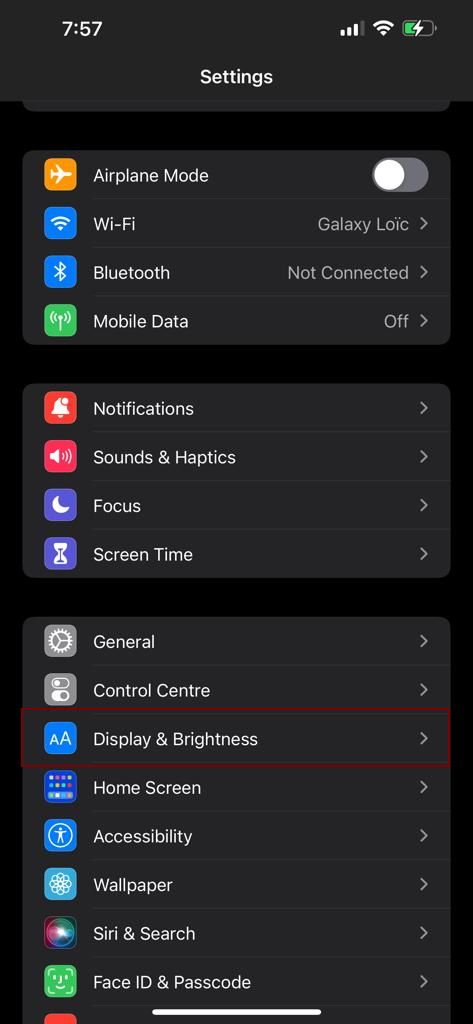A detailed phone screenshot captured at 7:57 shows the settings menu with a black and gray background. The menu options are presented within small gray bars, contrasting against the primary black background. The status indicators at the top reveal three bars of signal strength, active Wi-Fi, and a battery at half capacity.

From top to bottom, the options displayed are:
- Airplane Mode: Off
- Wi-Fi: Connected to "Galaxy Loic"
- Bluetooth: Not connected
- Mobile Data: Off

Further down, the settings include:
- Notifications
- Sound and Haptics
- Focus
- Screen Time
- General
- Control Center
- Display & Brightness (highlighted with a red border)

Additional options include:
- Home Screen
- Accessibility
- Wallpaper
- Siri & Search
- Face ID & Passcode

Each setting is accompanied by a right-facing arrow, indicating the availability of a sub-menu or further options. The mix of gray bars against the black background and the use of icons for each setting provides a clean and intuitive interface design.